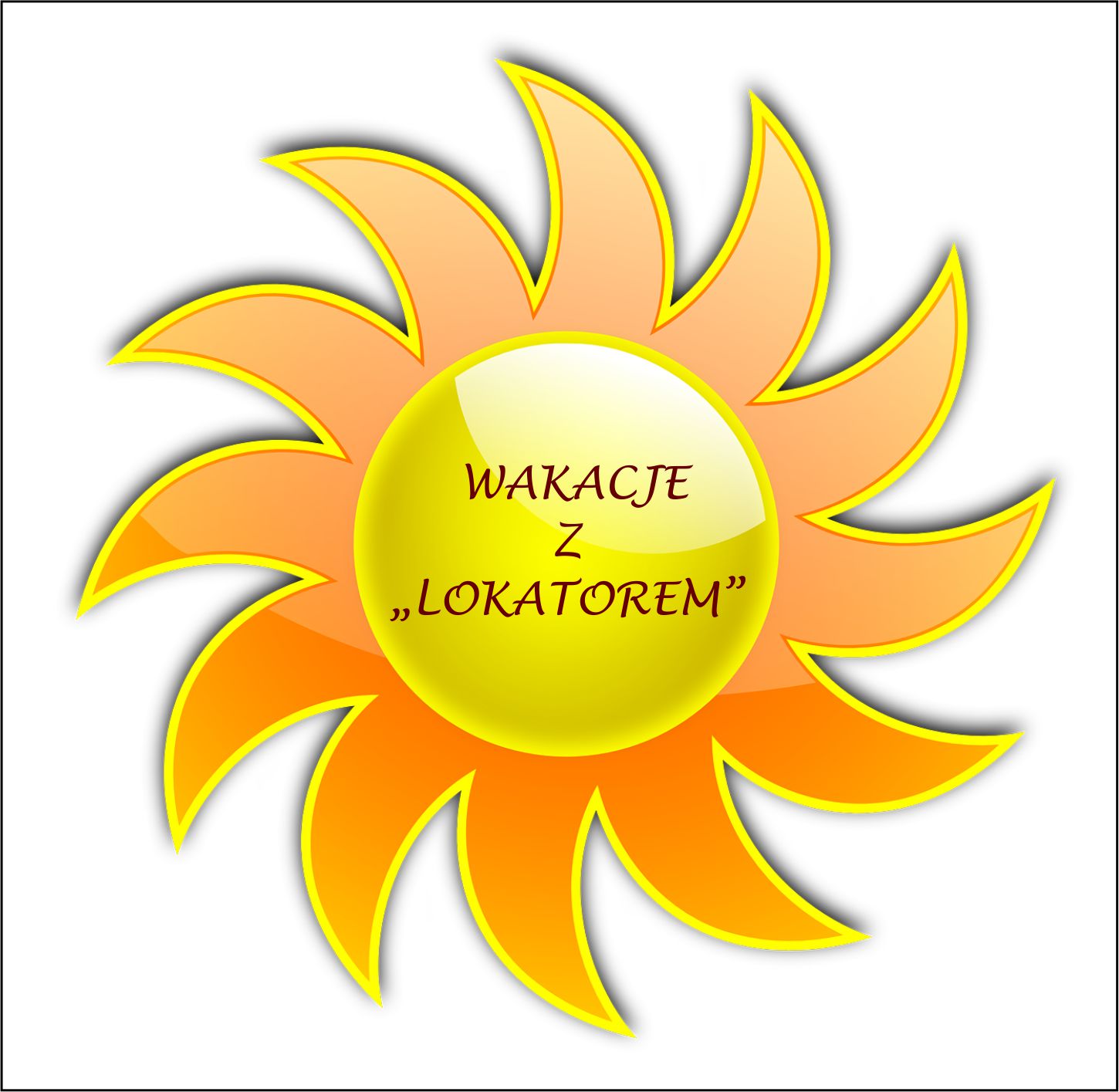This vibrant image features an abstract illustration of the sun, centered within a black-outlined square on a plain white background. The sun itself has a bright yellow center and is surrounded by orange, somewhat symmetrical spiraling 'flames' that typify a clipart style representation. Each flame is delicately outlined in a deeper yellow, mirroring the color of the sun's core. In the vertical middle of the sun's round center, there is brown text reading "Łakadzi Z Lokatorium,” suggesting a possible Polish phrase. This text is prominently enclosed in quotation marks, anchoring the composition with a focal point of linguistic intrigue.